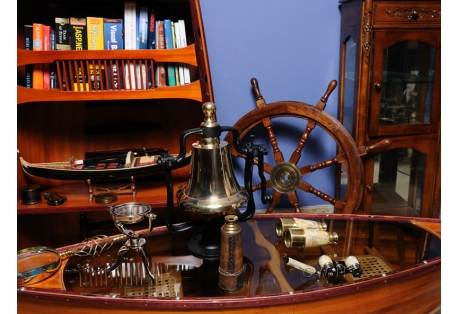This photograph captures a nautically themed family room, brimming with maritime charm. At the center of the room is a unique coffee table fashioned from brown wood with a glass top, resembling a canoe filled with various objects. Resting on the table are a large metallic bell, binoculars, a spyglass, and what appear to be smaller binoculars akin to opera glasses. This intriguing centerpiece sets the tone for the room’s decor.

Behind the coffee table stands a blue wall, enhancing the room’s cool, maritime ambiance. Against this wall is a wooden ship’s steering wheel, prominently placed between a slanted trapezoid bookshelf on the left and a wooden cabinet with glass panels on the right. The bookshelf is filled with books lined up on the top shelf, secured by a small wooden gate, while the lower shelf proudly displays a black canoe model, further emphasizing the nautical motif.

The wooden cabinet to the right, though only partially visible, adds a touch of elegance with its glass casings, the contents of which remain hidden from view. The overall setting is a harmonious blend of dark brown wooden furniture and maritime artifacts, creating a cohesive and visually captivating room.